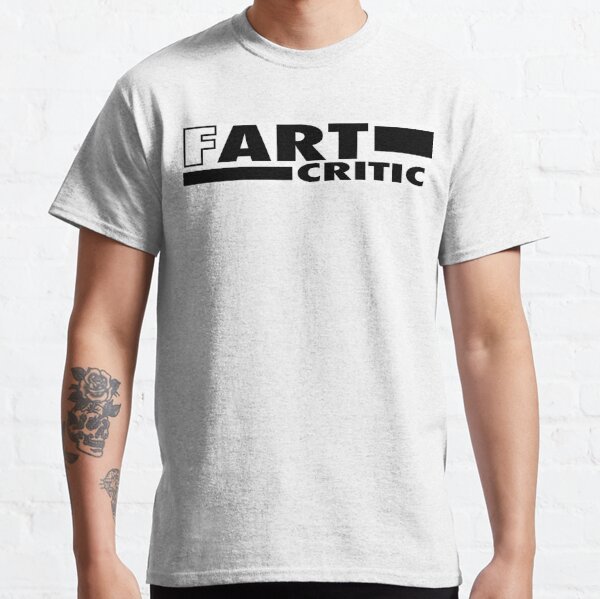The photograph depicts a vertically rectangular, full-color, indoor shot of a Caucasian male wearing a light-colored, short-sleeved t-shirt under artificial lighting. The background is a white-painted brick wall. The man’s face is not visible, only his neck and arms down to the wrists are shown. On his right forearm, there is a detailed black and white tattoo of a skull with a rose growing out of it, and there is another tattoo on the inner side of his arm. The t-shirt, predominantly light cream or white, has bold black text that humorously reads "F-ART CRITIC," with small dashes separating the "F" and "ART" and another dash after "ART."